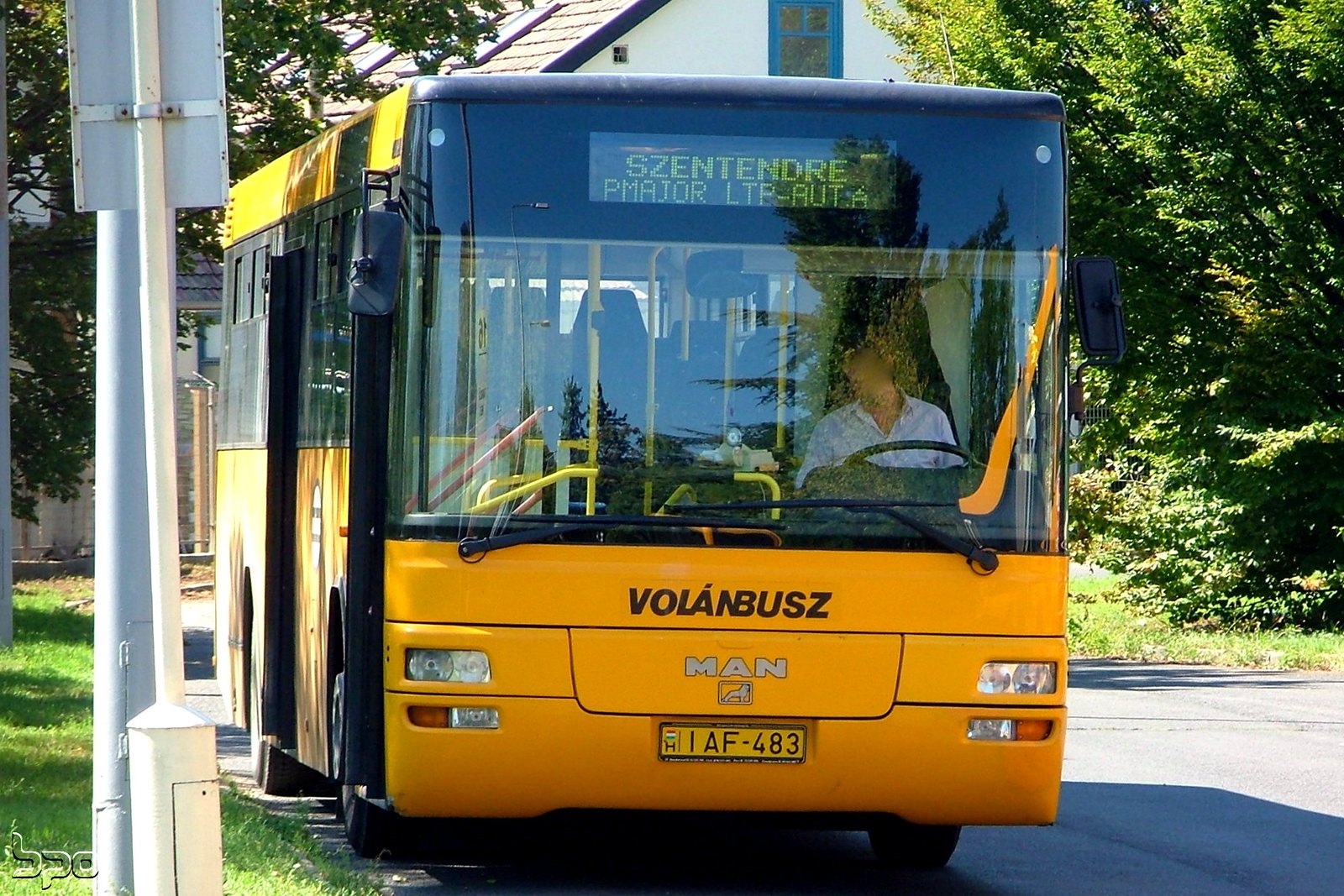This photograph depicts a bright yellow and black city bus, identified as a Volan Bus Man model, stationed at a bus stop in a verdant neighborhood, likely in a European city indicated by the digital readout text "Centendre Major LTP-AUTA." The front of the bus features a large picture window and has a license plate that reads "IAA." The bus is driven by a female driver, who appears to be checking a mirror inside the bus, possibly to monitor passengers. The driver is wearing a light blue or white shirt and has curly hair. Surrounding the bus, the scene comprises lush green grass to its left, asphalt and foliage to its right, and a white cottage-style house with an A-line roof behind it. Notably, the house features a blue-bordered window at the apex of the roof, adding a quaint charm to the backdrop. The neighborhood is lined with numerous trees, enhancing the overall greenery and serenity of the location.